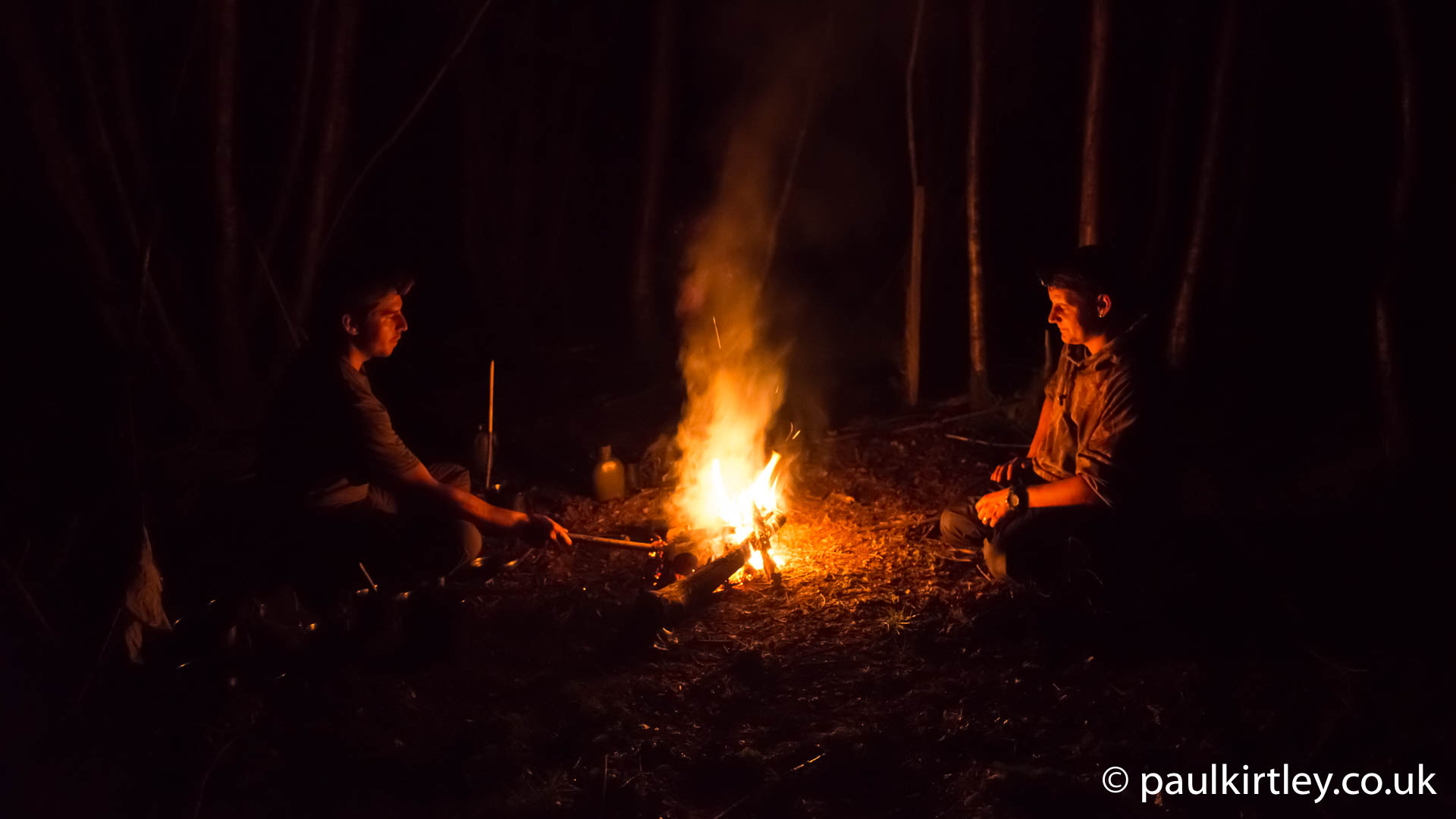This night-time photograph captures two young Caucasian men, aged approximately between 25 and 45, sitting on the ground in a dense forest illuminated by a bright campfire. The man on the left, seated cross-legged, is engaging with the fire using a stick held in his right hand, possibly stoking the flames or fidgeting with the burning logs, twigs, and branches. The man on the right, wearing a watch and sitting on his knees, is gazing directly into the fire, his face aglow with the fire's reflection. Both men’s brown hair and white skin are clearly visible in the intense light of the campfire, which is the sole source of illumination against the inky blackness of the surrounding woods. Behind them, faintly lit tree trunks and branches add depth to the dark background. The ground around them appears to be mostly dirt with scattered rocks, further illuminated by the fire's light. In the bottom right corner of the photograph, the text "paulkirtley.co.uk" along with a copyright symbol can be seen, and behind the man on the left, there appears to be a white bag or similar item.